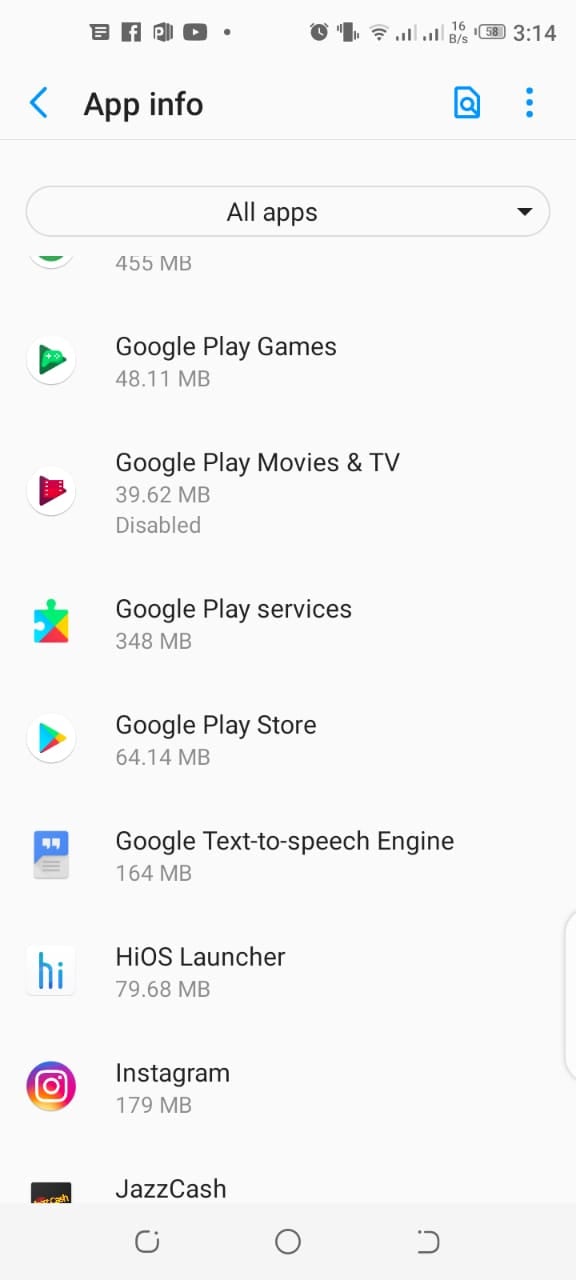This screenshot captures the app info section of a mobile phone. Displayed prominently at the top right corner, the current time is 3:14 PM, indicated alongside a battery icon showing 58% charge. Other status icons visible include an alarm clock, a vibrate icon, two cell phone signal strength indicators, and a 16 kbps data icon.

The central part of the screenshot reveals detailed information about various apps installed on the device, listed sequentially along with their respective storage sizes and icons. The list includes:

- **Google Play Games**: 48.11 MB
- **Google Play Movies & TV**: 39.62 MB (disabled)
- **Google Play Services**: 348 MB
- **Google Play Store**: 64.14 MB
- **Google Text-to-Speech Engine**: 164 MB
- **HiOS Launcher**: 79.68 MB
- **Instagram**: 179 MB
- **Jazz Cache**: (No size listed)

Each app entry is accompanied by its unique icon, such as a jigsaw puzzle piece for Google Play Services, a right-pointing triangle for the Google Play Store, and a document symbol for the Google Text-to-Speech Engine. The overall design is typical of mobile app management screens, providing an easily navigable interface for users to monitor and manage their app data usage.